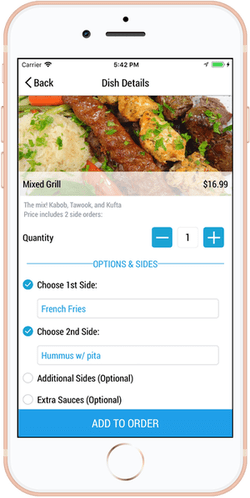The image depicts a smartphone with a pink edge and white cover. The screen displays an online food ordering interface, showing details for a dish called "Mixed Grill," priced at $16.99. The screen includes a blurry description of the dish. 

There are options for adjusting the quantity with a blue square button featuring a minus sign and another square button with a plus sign, with the number one displayed between them. Below, in blue text, it says "Options at Sides," followed by instructions in black text to "Choose one side." One option listed is "Fresh Fries" in a blue box.

Additionally, it allows the selection of a second side, with an option for "Hummus with Pita" displayed in a box. Beneath this, the interface offers "Additional Sides" and "Extra Sauces" as optional items, each with a corresponding circle for selection. At the bottom of the screen is a blue button labeled "Add to Order."